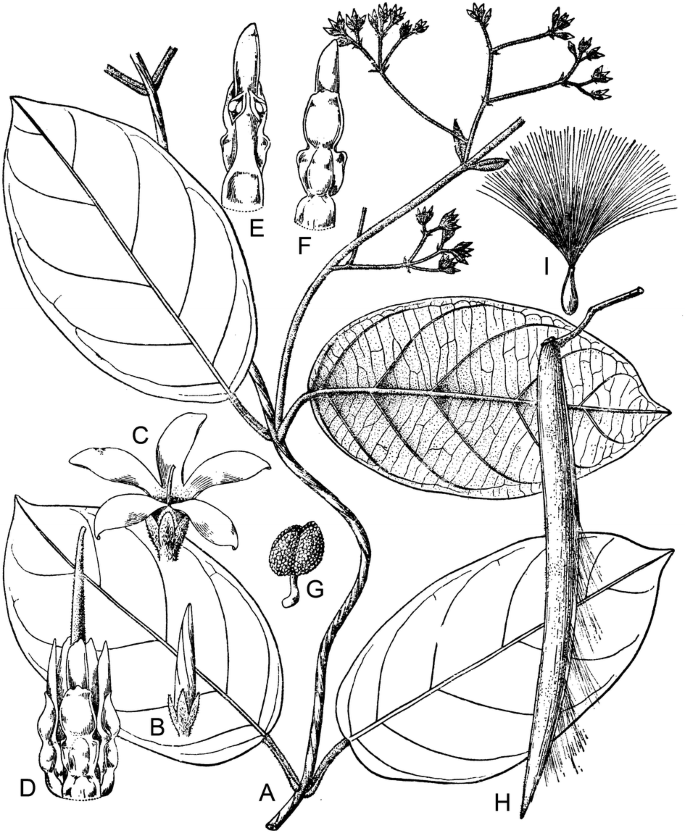This black-and-white pencil sketch depicts a detailed botanical diagram, primarily featuring various parts of a plant. The illustration is stark with dark pencil lines on white paper, showcasing intricate elements labeled with black, capital letters from A to I. At the base of the diagram, the main stem starts with label A and intertwines upward through the center of the image. Along this stem, a series of components branch out, including several ovate leaves, each labeled respectively. Notably, a leaf by the letter B, another near D, a flower with petal-like structure marked as C, and yet another leaf next to the letter H. To the right, a disconnected leaf with the letter G is observed. The structure marked I at the top resembles a fan, while near label H, a bean-like element–possibly resembling a vanilla pod–is drawn. Each part, meticulously labeled, suggests this illustration serves as a tool for identifying and studying the different parts of a plant.